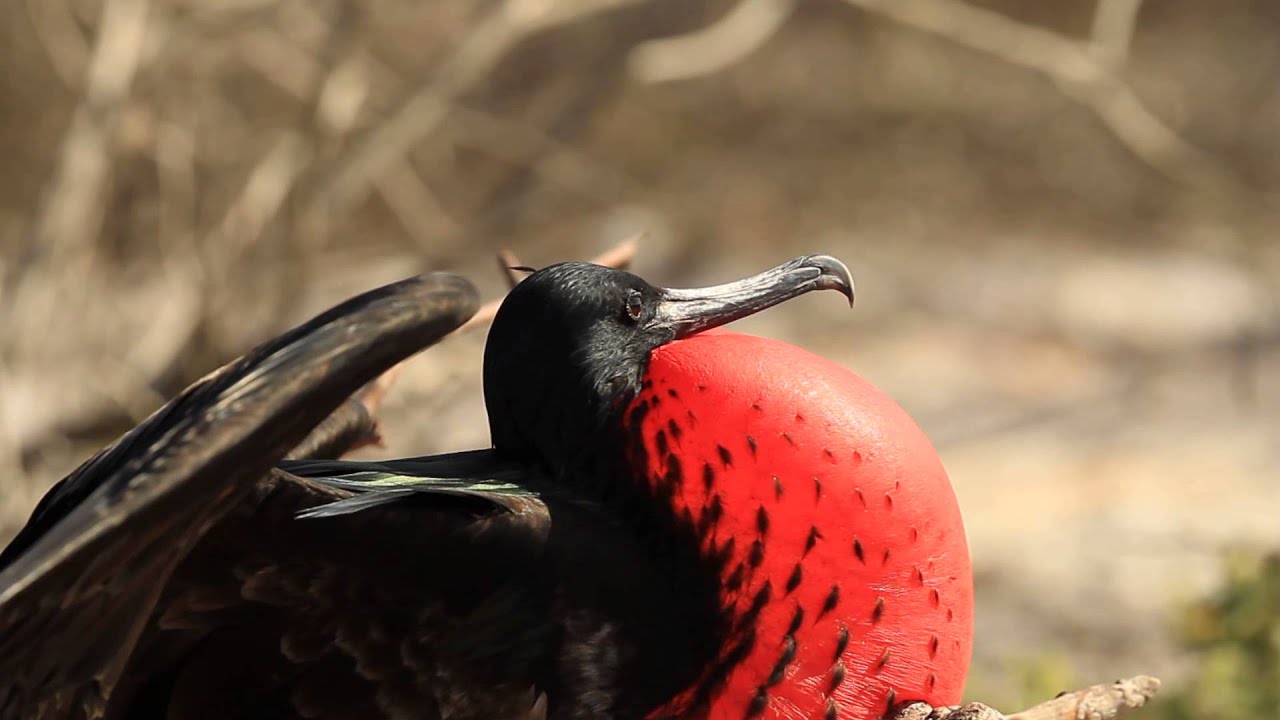The image portrays a detailed, close-up view of a unique bird species, prominently occupying the lower half and extending horizontally from the left-hand corner to past the middle of the image. The bird's striking features include a black head with a black eye, and a long, slender beak that is light gray at the base, darkening toward its curved, pointy tip. Its body, wings, and head are predominantly black, with the wings displaying some brown at the tips. The most distinctive characteristic of the bird is its bulging, frog-like red chest, resembling an inflated balloon with small black feather lines. The background of the image is blurry brown, with sticks visible in the upper left corner and some green in the bottom right, enhancing the natural setting. The overall image is bright and clear, capturing the bird in natural lighting.